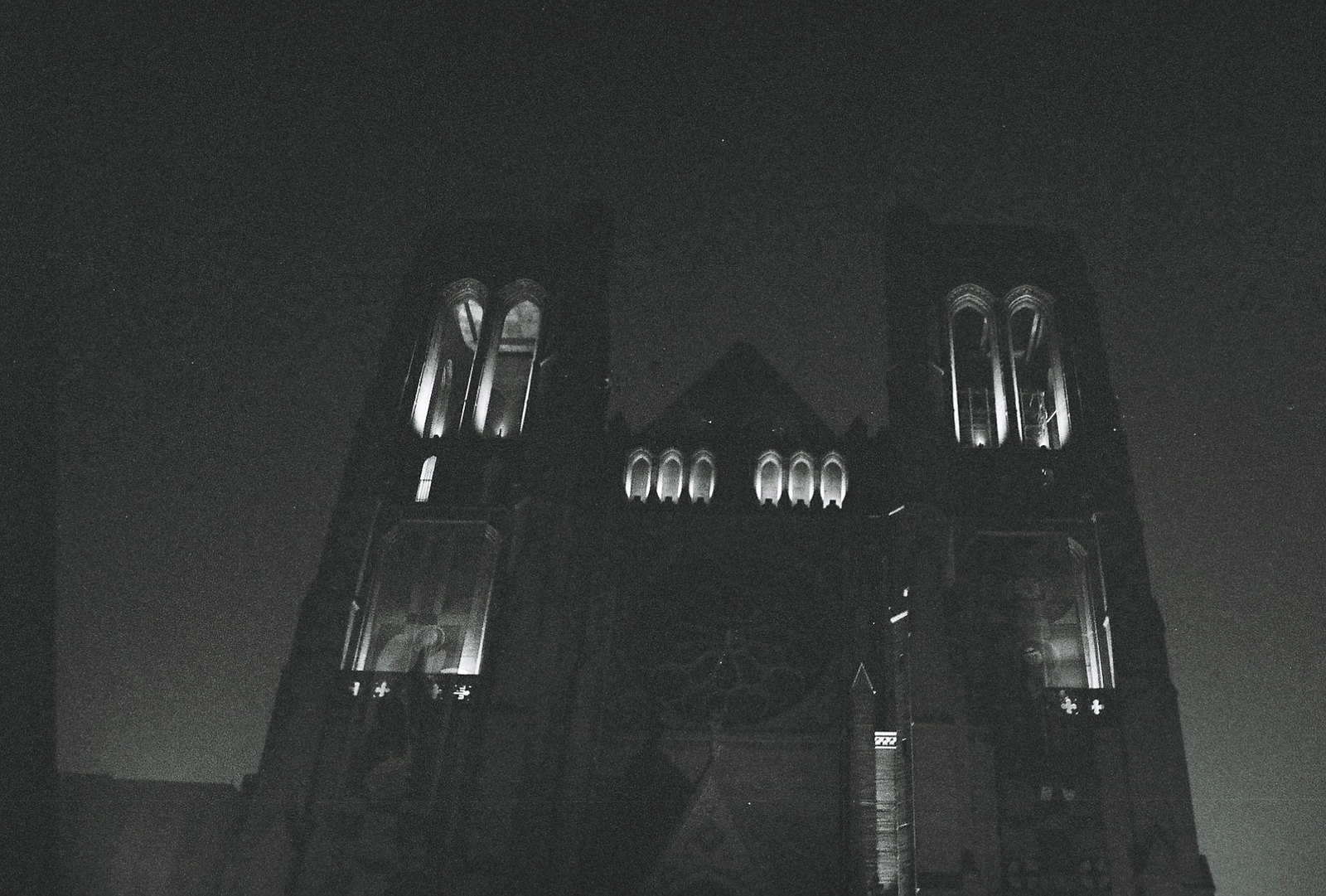This is a black and white nighttime photograph of an old, likely Catholic, cathedral. The image showcases a dark, possibly intimidating atmosphere with no people present. The cathedral features two prominently illuminated towers on the left and right sides, each adorned with partially open, large oval or oblong windows that might serve as bell towers. Between these towers, a shorter central steeple with a triangular roof stands out. The façade includes a large, round stained glass window in the center, above a set of two square windows. Additionally, six small arched or rounded windows line the walkway area, their soft luminescence adding to the eerie beauty. The overall composition lacks text, dates, or names, highlighting the architectural details and the interplay of light and shadow.